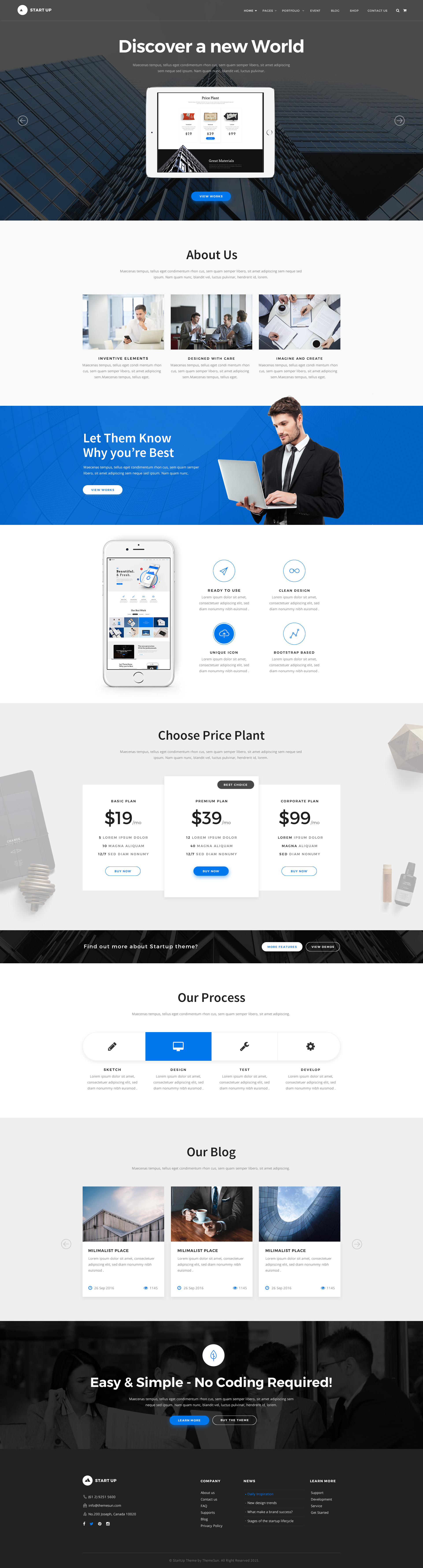The image features a complex layout starting from the top where a black border contains the text "Discover a New World." Directly beneath this, there is a white box housing various icons. The next section features a white background with three small, indistinct thumbnails; though the details are unclear, they appear to depict people.

Further down, a blue box with text is visible, next to which is an image of a man in a business suit examining some documents. Right below this, there is a picture of a screen accompanied by some text. The following section has a gray background with several white boxes, each containing text and pricing information: $19.00 in the first box, $39.00 in the middle, and $99.00 in the rightmost box.

Moving further down, there are three additional small thumbnails with a blue box positioned above them. At the very bottom of the image, another black border is present, displaying large white letters at the top and a smaller blue button situated underneath.